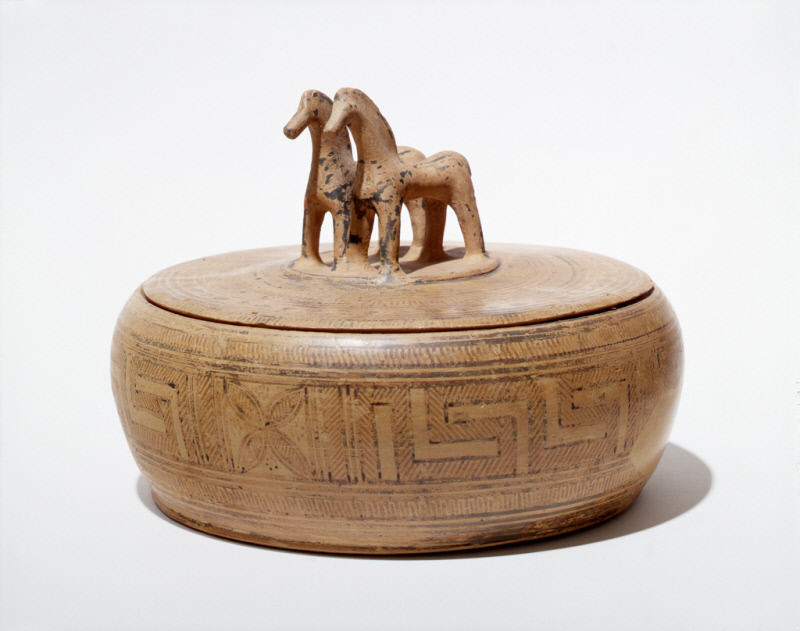The image is a rectangular landscape photograph depicting a small, round container crafted from clay or pottery, possibly with an antiquated or museum-like quality. The container features a tapered base that broadens towards the top before becoming smaller again and is adorned with intricate maze-like patterns and etchings, including flowers, diagonal lines, and L-shapes in black and tan hues. The orangey salmon-colored piece, showing signs of wear with black spots, is capped with a slightly open lid in a matching color and style. This lid serves as the base for two rusted statues of horses facing left and down, which also act as a handle, casting a shadow to the right of the container.